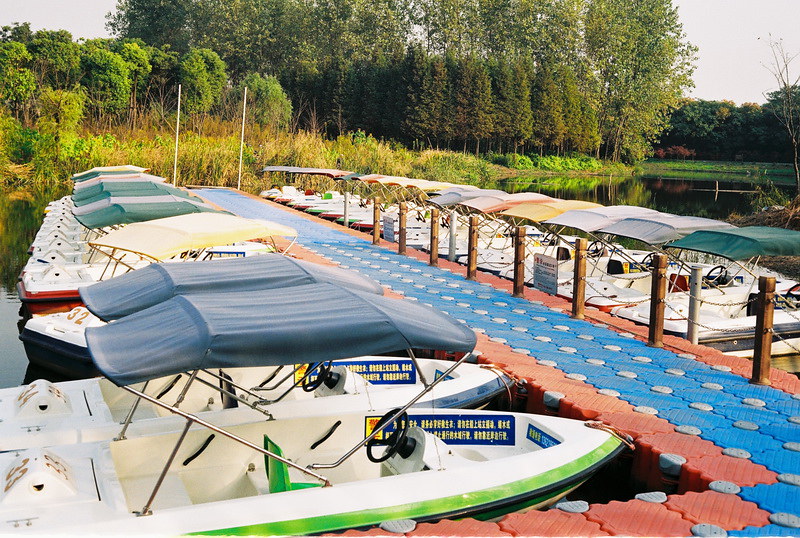This photo depicts a vibrant boat dock set against a swampy, lush green backdrop. The dock, made of interlocking plastic tiles, features a striking combination of blue and pink panels bordered with red and gray grip circles. Moored along both sides of the dock, there are numerous small, white boats with fabric canopies supported by silver steel poles. Each boat is designed to hold one to two passengers and has identifiable numbers on their backs, such as 32, 33, and 34. Some boats even display stickers or instructions likely meant for rental purposes. The dark and murky water surrounding the dock exudes an air of mystery, mirroring the dense forest of tall, green trees and a grassy hill in the distance. This picturesque scene suggests a tranquil yet intriguing recreational spot, framed by nature's lush beauty and the stillness of the water.